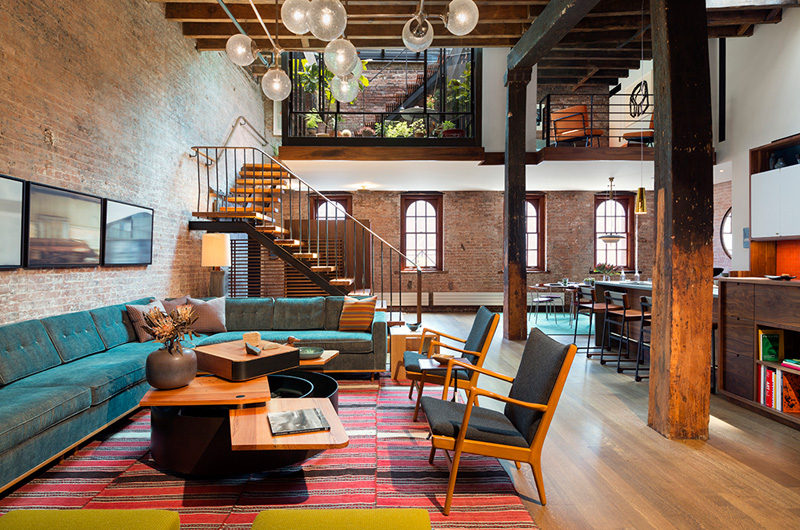The image showcases the interior of a spacious house with an open floor plan. The floor is made of medium brown hardwood tiles, visible at the lower right corner of the picture. Dominating the left side of the room is a large area rug composed of various sections with a striped pattern in black, white, and red. Centered on this rug is a wooden coffee table, flanked by wooden chairs on the right and a sizeable curved sectional sofa on the left. The sofa features bluish-green cushions adorned with throw pillows.

A prominent vertical wooden beam stands in the middle of the image; its color transitions from brown at the base to black at the top. Behind the sofa, a staircase with a metal railing ascends to a visible second floor. The stairs initially rise to the left before turning right at a landing. The second floor has a large window and appears to extend to an outdoor area with plants.

Further adding to the room's character are large wooden posts and a big brick wall. Hanging frosted white lights illuminate the room, and rounded-top windows on the lower level provide additional natural light. The overall decor suggests a cozy and stylish living space.